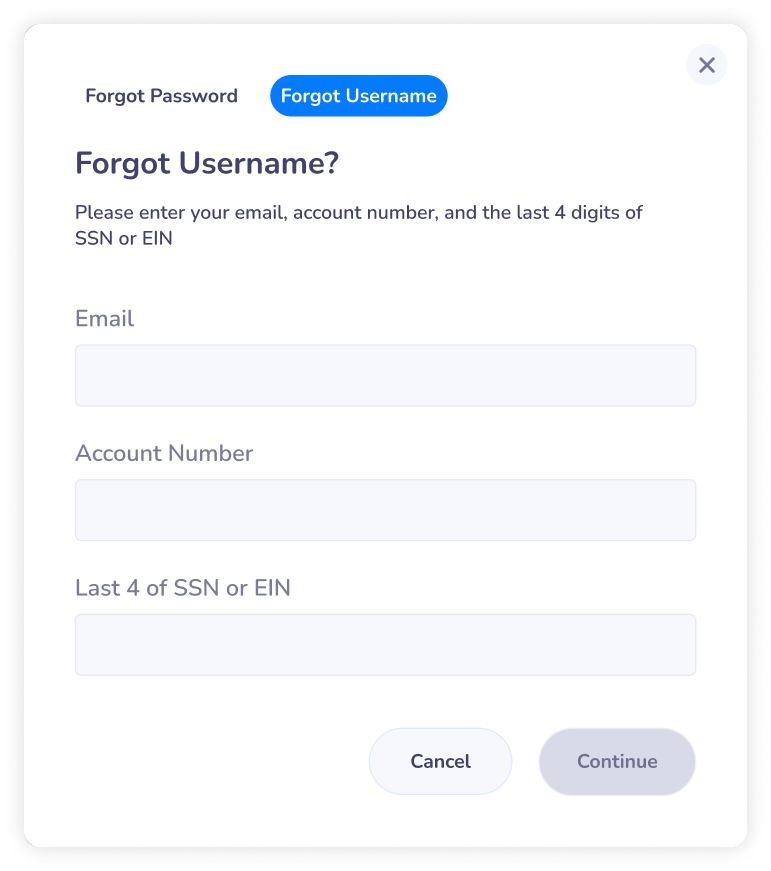The image depicts an account recovery form designed to help users retrieve their forgotten username. The form is set against a white rectangular background that is taller than it is wide. 

In the upper left corner, bold black text reads, "Forgot Password?" Beneath this text, there is a prominent blue button with white text that says, "Forgot Username?"

Below the button, the form instructs users with the text: "Please enter your email, account number, and the last four digits of your SSN or EIN."

The form consists of the following fields:
1. **Email:** Accompanied by an empty data field.
2. **Account Number:** Followed by another data field.
3. **Last Four of SSN or EIN:** With a corresponding data field.

At the bottom right corner of the form, there are two buttons. The first is a white "Cancel" button with gray font, followed by a gray "Continue" button with darker gray text.

The primary colors utilized in the design are white, black, blue, and various shades of gray. The form appears to be part of a password or username recovery process, aiming to assist users in retrieving their username. There are no distinct logos or other branding elements that relate to a specific account or service.